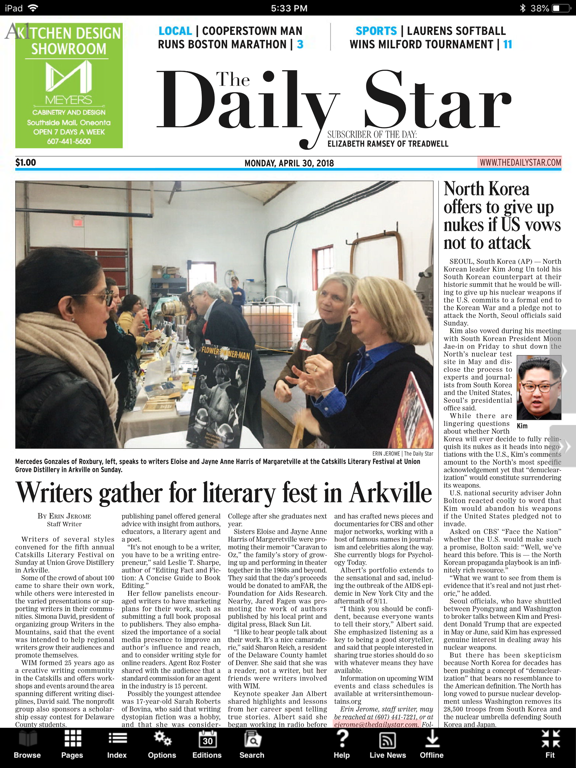The image displays the front page of the Daily Star newspaper, viewed on an iPad at 5:33 p.m. with the device's battery at 38%. The edition, priced at $1, is from Monday, April 30th, 2018. The masthead prominently reads "The Daily Star," with a subheading announcing "Subscriber of the Day: Elizabeth Ramsey of Treadwell." In the top left-hand corner, a green box advertises "Kitchen Design Showroom, M for Myers."

Above the newspaper's title are two section headings: "Local: Cooperstown man runs Boston Marathon on page 3" and "Sports: Lauren Soppel wins Milford tournament, page 11." The main feature image below these headings captures a bustling literary festival in Arkville. The scene depicts authors engaging with attendees over tables, set in what appears to be a garage or barn. The caption for the image reads, "Writers gather for literary fest in Arkville." To the right of the main article, a sidebar features a photo of Kim Jong Un, accompanied by the headline, "North Korea offers to give up nukes if US vows not to attack."